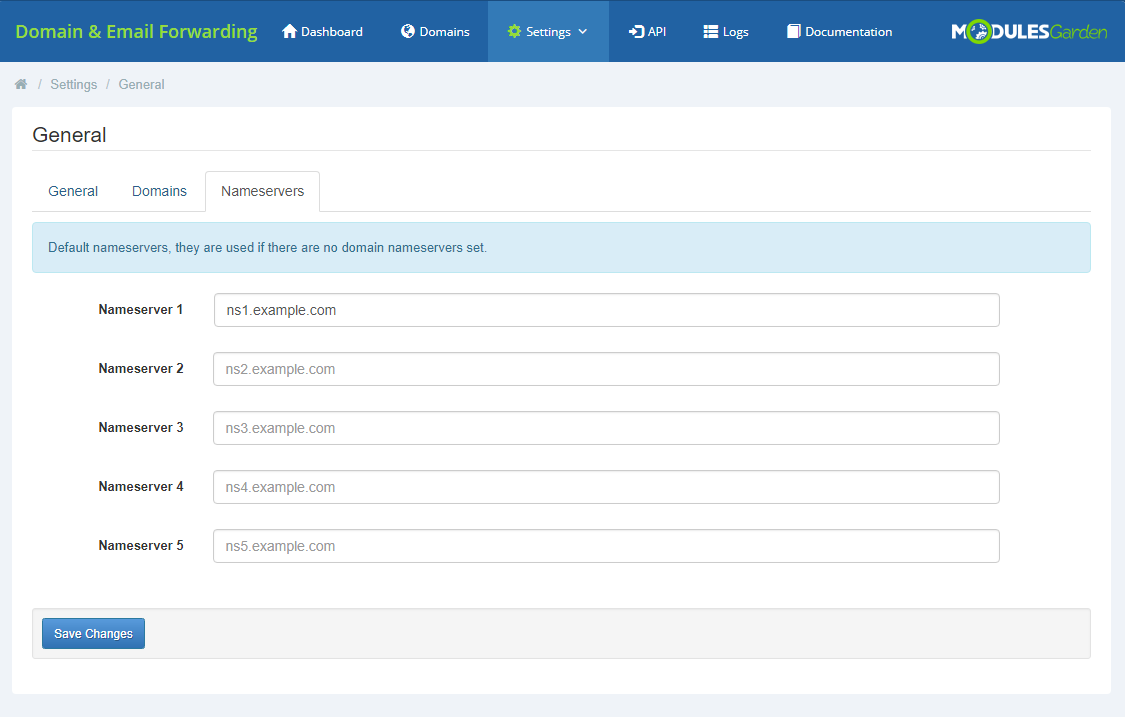Caption: 

The image displays a detailed form for domain and email forwarding set against a clean, white interface. At the top of the form, the section header "Domain and Email Forwarding" is highlighted in green, while key navigation options appear in white text: "Dashboard," "Domain Settings," "API Logs," "Documentation," "Modules," and "Garden." The main content area is divided into three sections, with the "General" category currently expanded, specifically focusing on "Domains and Name Servers."

Within this focused section, instructions and fields for configuring name servers are provided. Detailed descriptions indicate that default name servers will be used in the absence of custom configurations. The form includes five name server fields already populated with URLs: 
- Name Server 1: ns1.example.com
- Name Server 2: ns2.example.com
- Name Server 3: ns3.example.com
- Name Server 4: ns4.example.com
- Name Server 5: (another field ready for input)

In the bottom left corner of the form, there is a prominent blue "Save Changes" button, allowing users to submit their configurations.